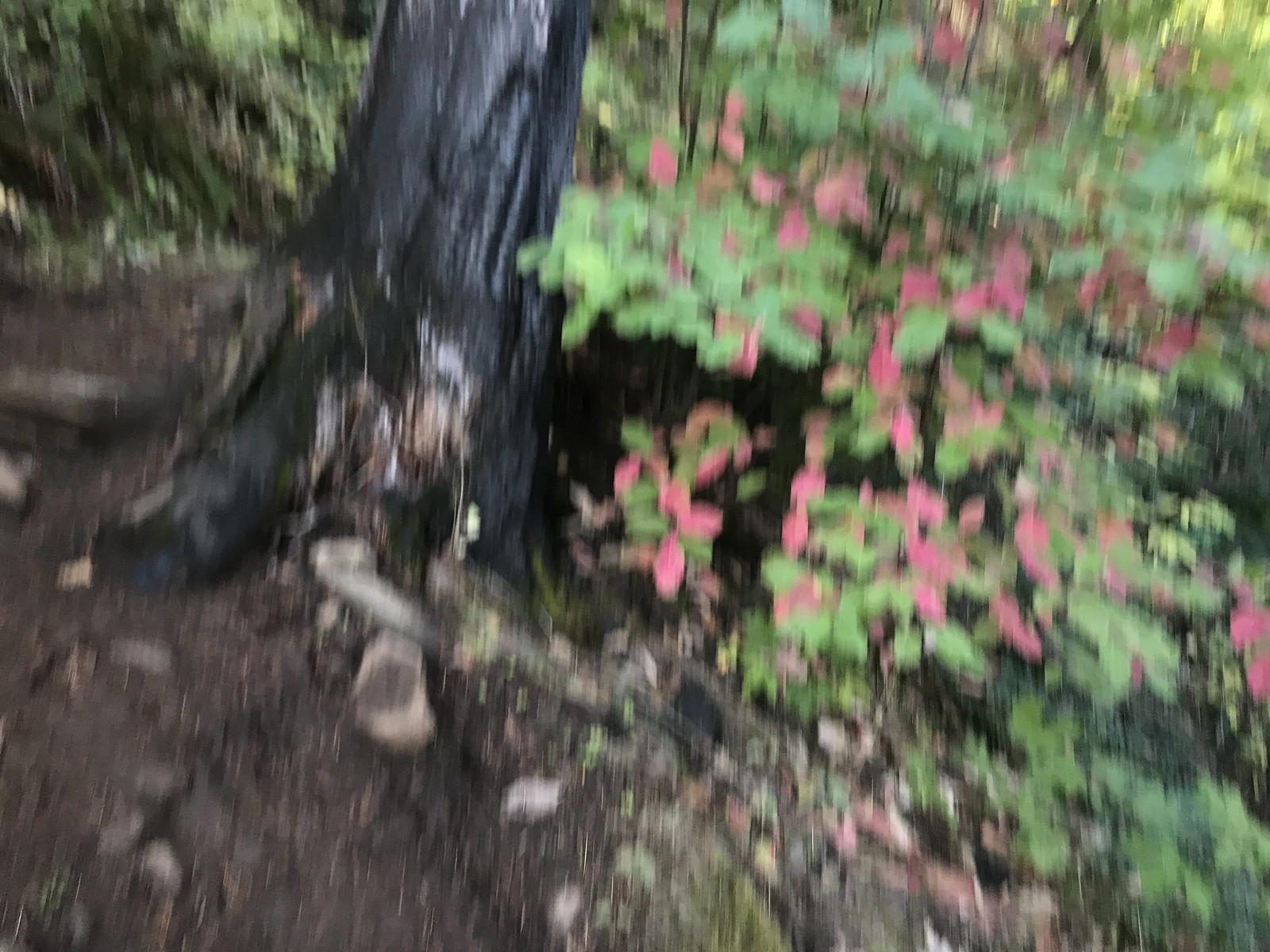This is a highly blurred photograph of an outdoor scene featuring a prominently dark and thick tree trunk, possibly blackened by a recent fire or darkened due to wet conditions. The base of the tree shows twisted roots embedded in almost black or very dark brown soil. Surrounding the tree trunk, there are patches of bare dirt and some green foliage. On the left side, there are green leaves supplemented with what appear to be pink or light purplish leaves or flowers, though the poor image quality makes it difficult to ascertain. The background reveals signs of new growth with dense shrubbery and additional foliage, suggesting a recovering natural environment. The scene appears to be sunlit, indicating it was taken on a sunny day. Despite its blurriness, the photograph captures the juxtaposition of charred remains and emerging life.